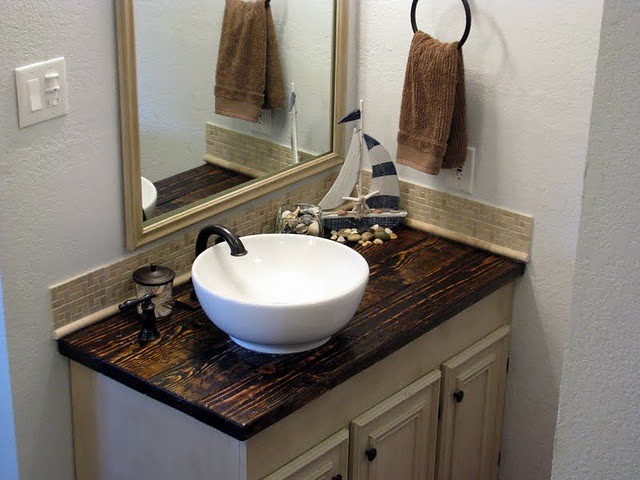The bathroom features a textured, white wall that serves as a backdrop for the various elements on the counter. On the left side, there's a light switch, followed by a gold-framed mirror mounted on the wall. Adjacent to the mirror, a towel ring holds a brown hand towel. Below that, a light brown tiled backsplash contrasts with the thick, dark wooden countertop of the sink area. The sink itself is a striking bowl design in white, paired with a sleek black faucet. Decorative elements include a nautical-themed sailboat with blue and white stripes, a starfish, and a small glass container filled with shells. Beneath the wooden countertop, beige-brown cabinets with circular brown handles provide storage and balance the aesthetic of the room.